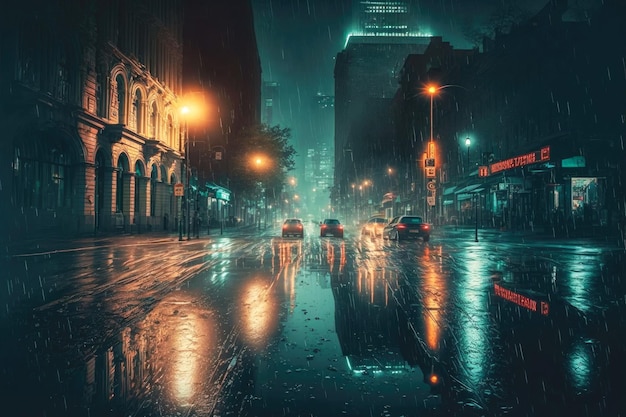This image captures a rainy night in a bustling urban city, filled with a palette of dark bluish-green hues and contrasted by the warm yellow of streetlights. The wet streets in the center of the scene reflect the surrounding buildings and lights, creating a glossy, mirror-like effect. On the left side, brown brick buildings and streetlights softly illuminate the area, while the right side features vibrant neon signs and a particularly tall building emitting light from its upper windows. The farther back in the image, there are cars with illuminated taillights visible, driving through the wet streets. Large, prominent buildings, potentially including an iconic structure resembling the Empire State Building with its top lights glowing, dominate the background. Trees line the left side of the picture, adding a touch of nature amidst the urban setting. The overall ambiance is a blend of calmness and quietude, punctuated by the reflections of city lights on the rain-soaked streets.